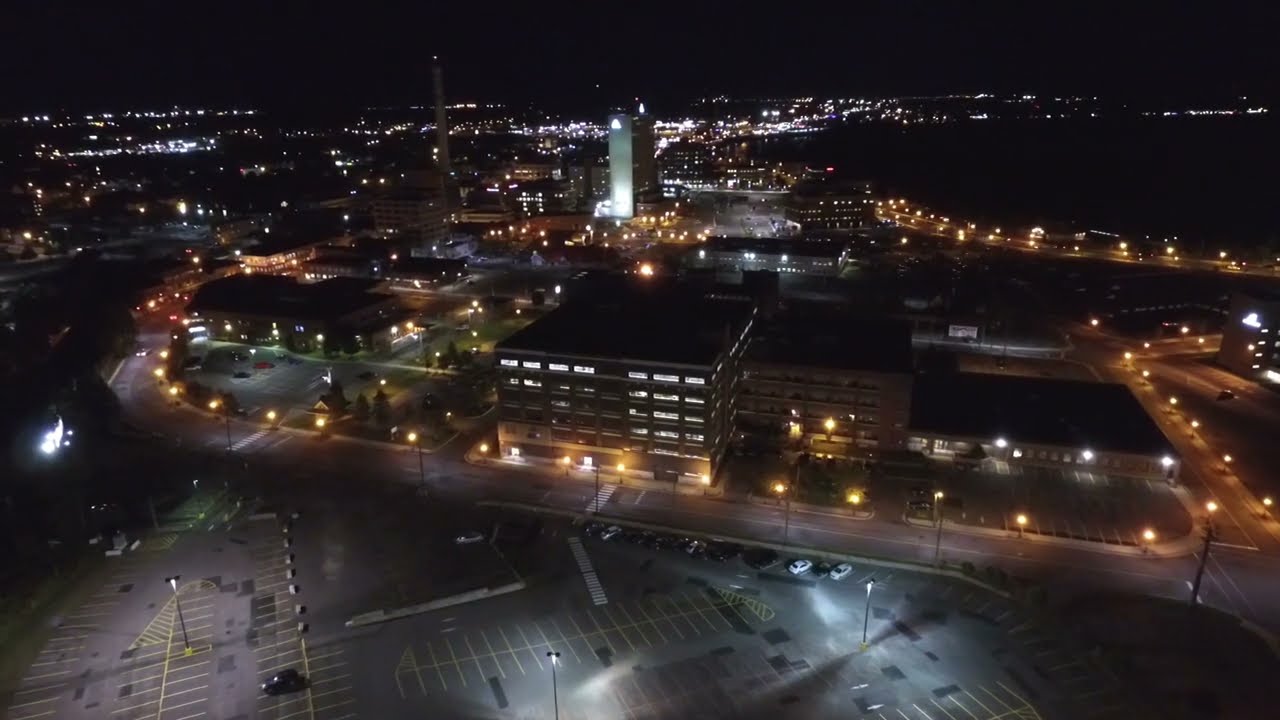The image captures a nighttime cityscape featuring a large, predominantly empty parking lot in the foreground, which spans across the bottom edge of the photo. The parking lot, illuminated by streetlights, has several cars scattered around its perimeter. Directly in the center of the image stands a large, multi-story building, possibly a parking garage, hospital, or hotel, with roads lined by lights surrounding it. Skyscrapers of varying heights can be seen in the distance, their lights blending into a colorful blur against the dark, black sky. The scene is well-lit with streetlights, and a few vehicles navigate the roads with their headlights on, highlighting what appears to be a fairly quiet but brightly illuminated urban nightscape.